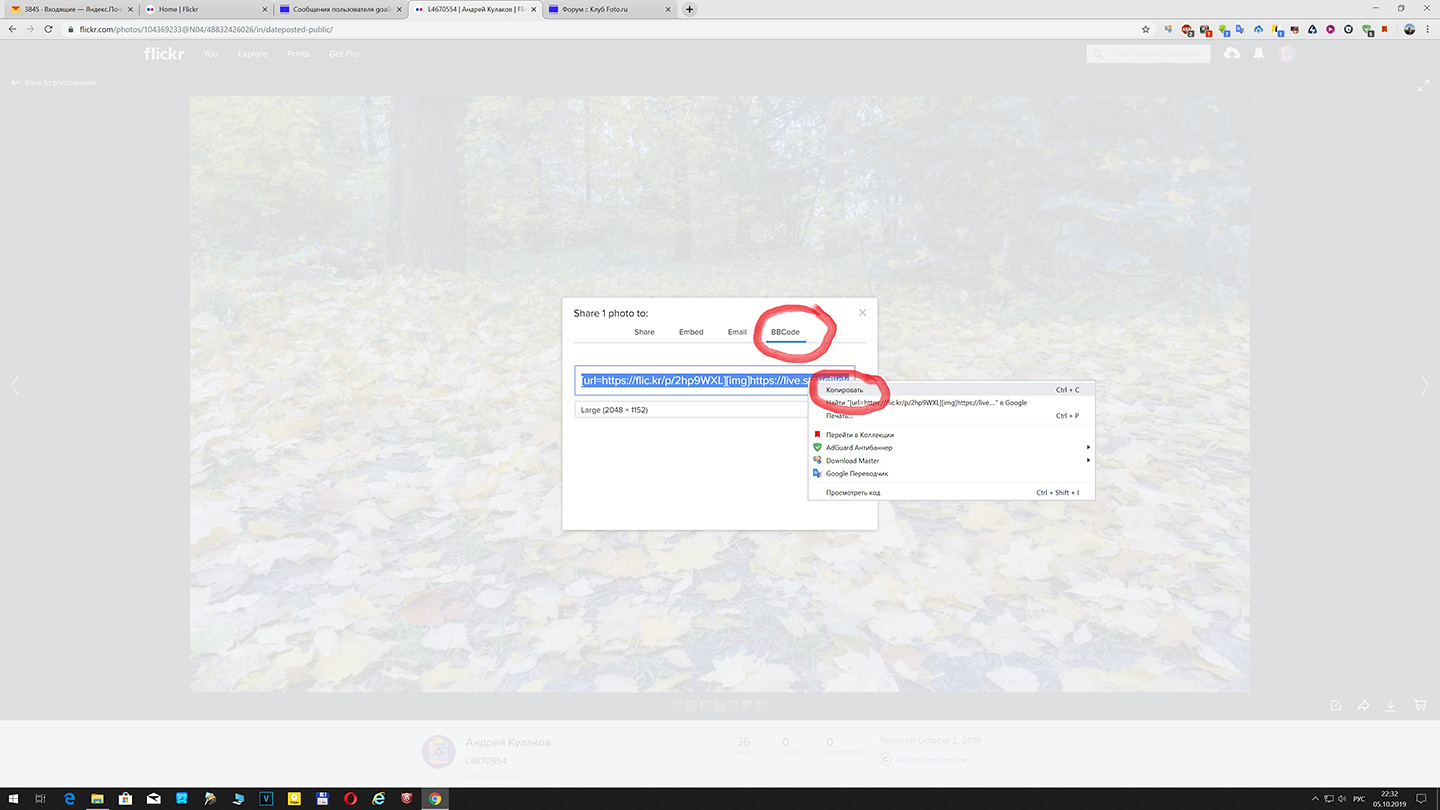The image showcases a computer screen with approximately five tabs open at the top, with Flickr.com being the currently active site. Two distinct open windows are visible; one displays options titled "Share," "Embed," "Email," and "BB Code," alongside the image size "Large 2048x1152." Adjacent to this window is another section containing various writings, some in Russian and some in English, including the term "Download Master." 

The screen's bottom features a taskbar with around 15 clickable application icons, spanning from Google Chrome and Internet Explorer to a folder icon, all positioned along a black line. The desktop background behind these elements depicts a grainy, blurred image of a forest with trees.